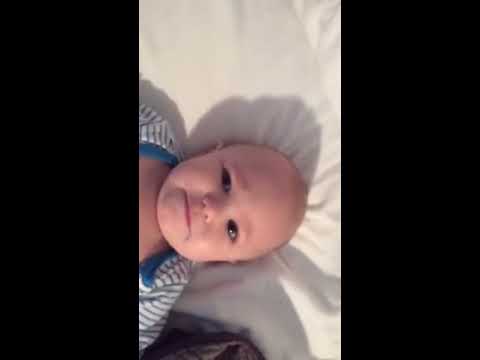This vertical image captures a baby lying sideways, as if it were a screen grab from a video. The baby, with a neutral expression and blackish eyes looking directly into the camera, is bald and has a slight shine on its right cheek, hinting at the light source. The infant is dressed in a white and blue striped onesie with a white collar, and is lying on a white pillow, which has a shadow cast by the baby's head. The scene is framed with thick borders on the left and right sides, creating a central focus on the baby. At the bottom left of the image, a small gray object, possibly the edge of a backpack, is slightly visible. Overall, the image is devoid of other elements except for the dark borders and the baby lying on what appears to be a white crib mattress.